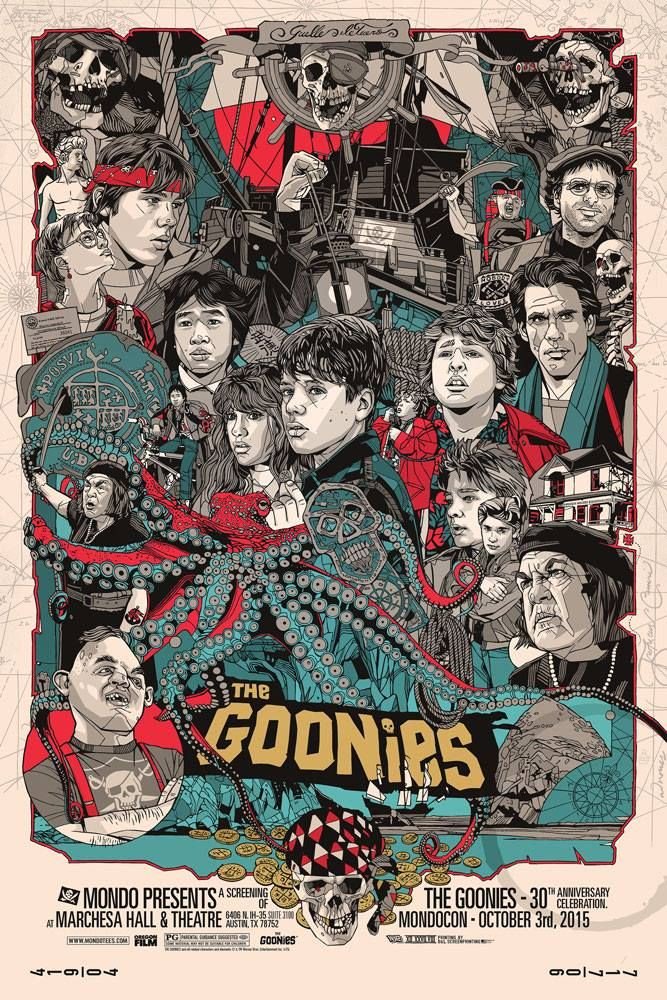The poster for "The Goonies" movie, presented in a visually striking collage style, showcases various characters from the film artfully drawn with intricate pencil work that lends a realistic texture to their faces. Dominating the center is a colossal octopus, its form highlighted with reddish and blue hues, contrasting with the primarily black and white composition of the poster. Interwoven in this bustling collage are a series of artifacts, including gold coins, a bandana-clad skull, a pirate ship, and even appearances by iconic imagery such as Michelangelo’s David. The characters, shaded mostly in gray tones, surround these vibrant elements, creating a dynamic and engaging scene.

At the lower center of the poster, the movie's title, "The Goonies," is prominently displayed in pale yellow letters with the dot over the 'i' replaced by a small skull. Below the title, the poster further commemorates the film’s legacy with details like "30th Anniversary Celebration" and mentions of the event date, October 3rd, 2015. Additional fine print includes credits and the note "Mondo presents a screenplay," adding a layer of classic movie poster authenticity.